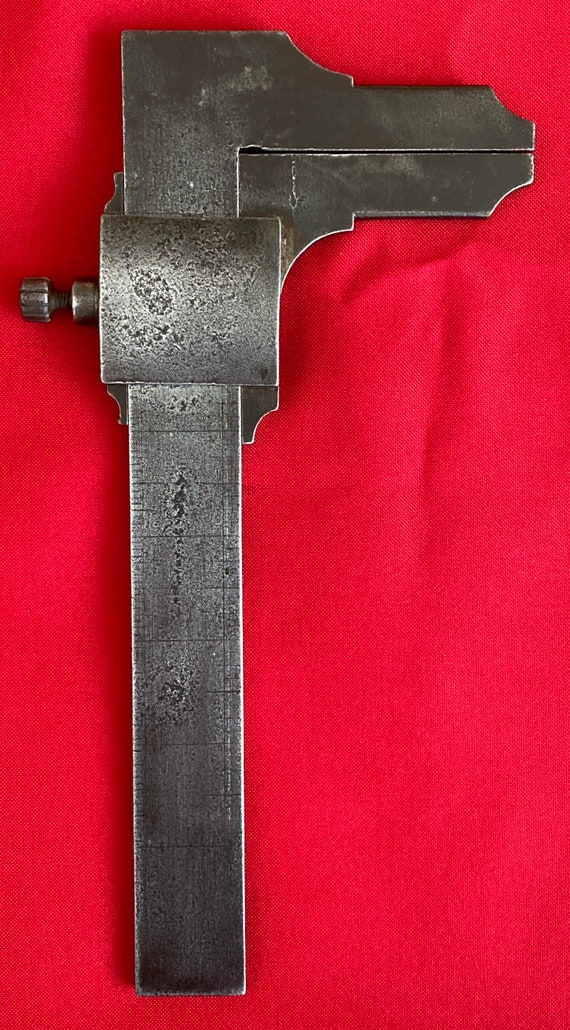This photograph features an old-fashioned caliper, likely made from iron or steel, characterized by its blackish-silver or brown-gray metal color. The caliper grippers are oriented to the right, with a small screw on the left side (from the viewer's perspective) that can be loosened to slide the jaw open and tightened to set the desired width. The caliper also includes a measuring scale along the handle, likely marked in increments similar to a ruler, though the markings are faint and difficult to read. This tool, looking quite aged, is lying on a red background that appears to be a piece of fabric, possibly a napkin, given its wrinkled texture. The setup provides a vertical presentation of the caliper, enhancing its vintage and utilitarian appeal against the vivid red fabric backdrop.